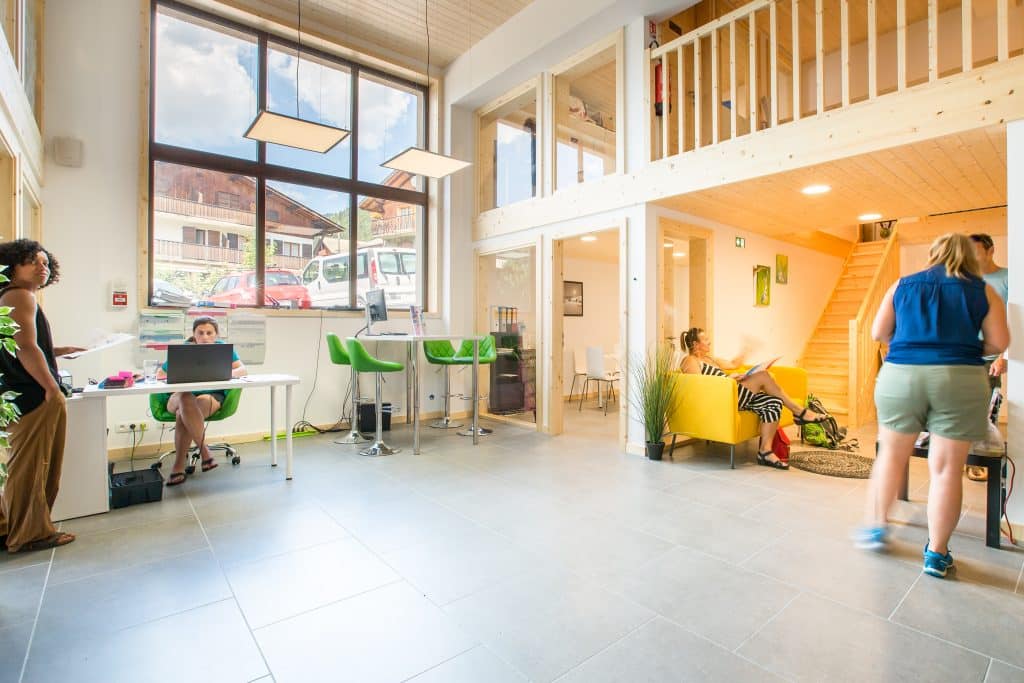The image depicts a spacious, modern workspace with a clean, minimalist design. The floor is composed of large gray tiles with white grout. On the left side of the image, a black woman with short hair, dressed in a black shirt, brown baggy pants, and sandals, stands looking to the right. Beside her is a rectangular white desk where a white woman in a teal shirt, shorts, and flip-flops sits cross-legged, working on a black laptop. The desk is pushed against the wall, over which six square windows with a view outside are arranged. Above her, two black poles descend from the ceiling, holding flat, rectangular lights with white faces.

Towards the center of the room, the scene transitions, featuring a modern kitchen island with bar stools that have silver bases and green cushion seats. Nearby, a white table with four green chairs sits close to the white wall. Moving to the right side of the image, the color palette becomes more varied. A large yellow armchair accommodates a woman in a black and white striped dress, while behind her, a wooden staircase ascends to a visible loft area in the upper right corner, outlined by a railing.

In the same section of the room, another woman stands with her back to the viewer. She wears a sleeveless blue shirt, green shorts, and blue tennis shoes, and she faces a man in a blue shirt. Both the design elements, including modern furniture and large windows, and the eclectic mix of people working, standing, and interacting, suggest a dramatized portrayal of a contemporary, versatile workspace, possibly styled for a promotional photo.